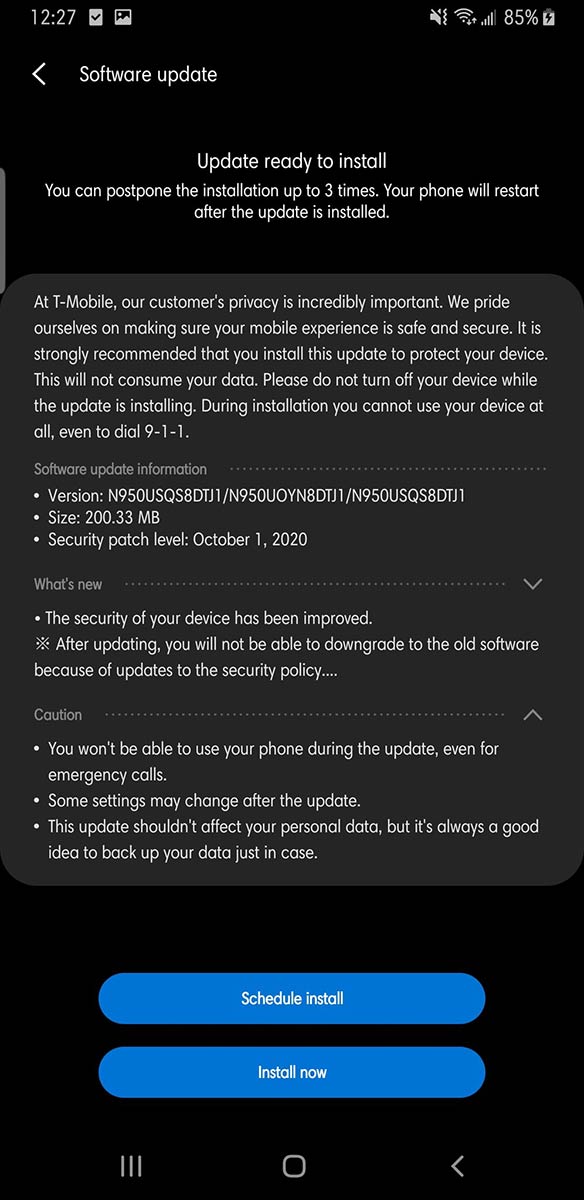This image is a screenshot of an Android phone's software update notification. The background is black, and the time displayed is 12:27. There is a notification visible, signaling a received image. The device is on vibrate mode, showing a high signal strength, with the battery at 85% and currently charging.

The notification is titled "Software Update" in white text. At the top, it states "Update ready to install," noting that the installation can be postponed up to three times. The phone will automatically restart after the update.

Below this, there is a message from T-Mobile emphasizing the importance of customer privacy and urging users to install the update for enhanced security. The message reassures that the update will not consume mobile data and advises users not to turn off the device during installation. It also highlights that the device will be unusable, even for emergency calls, during the update process.

Further down, detailed software update information is provided, including the version, size, and the last patch level date. The "What's New" section outlines the new features and improvements included in the update.

A cautionary note at the bottom reiterates that the phone will be unusable during the update and mentions that some settings may change. Although the update should not affect personal data, it is advisable to back up data just in case.

At the bottom, there are two blue oval buttons for user action: "Schedule Install" and "Install Now."